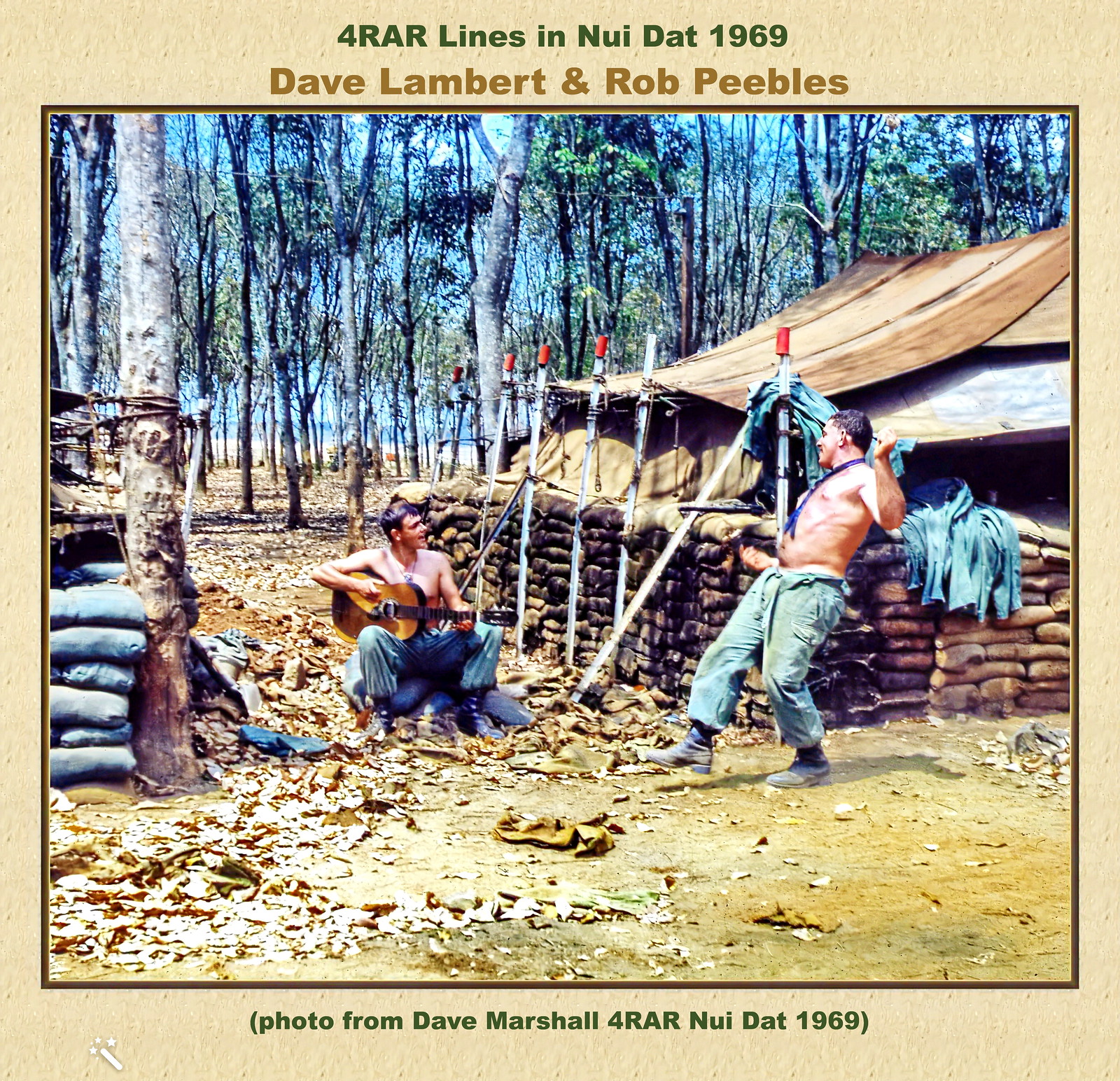Title: Four RAR Lines in New Dart 1969, Dave Lambert and Rob Peeples

Caption: In this evocative image titled "Four RAR Lines in New Dart 1969," featuring Dave Lambert and Rob Peeples, the scene is set against a backdrop of tall, densely clustered trees. Central to the composition is a man seated on a collection of blue bags, possibly sandbags, deeply engrossed in playing a guitar. Both men in the image are heavily attired, wearing blue pants. The second man, positioned to the right, leans slightly backward, appearing relaxed. Further to the right stands a rustic structure with a brown roof, enveloped by numerous brown bats. The setting appears to be in a wooded area, with logs and sticks scattered around, contributing to an earthy ambiance. A tent, held up by slender metal rods, is also visible amidst the trees, adding to the camp-like atmosphere.